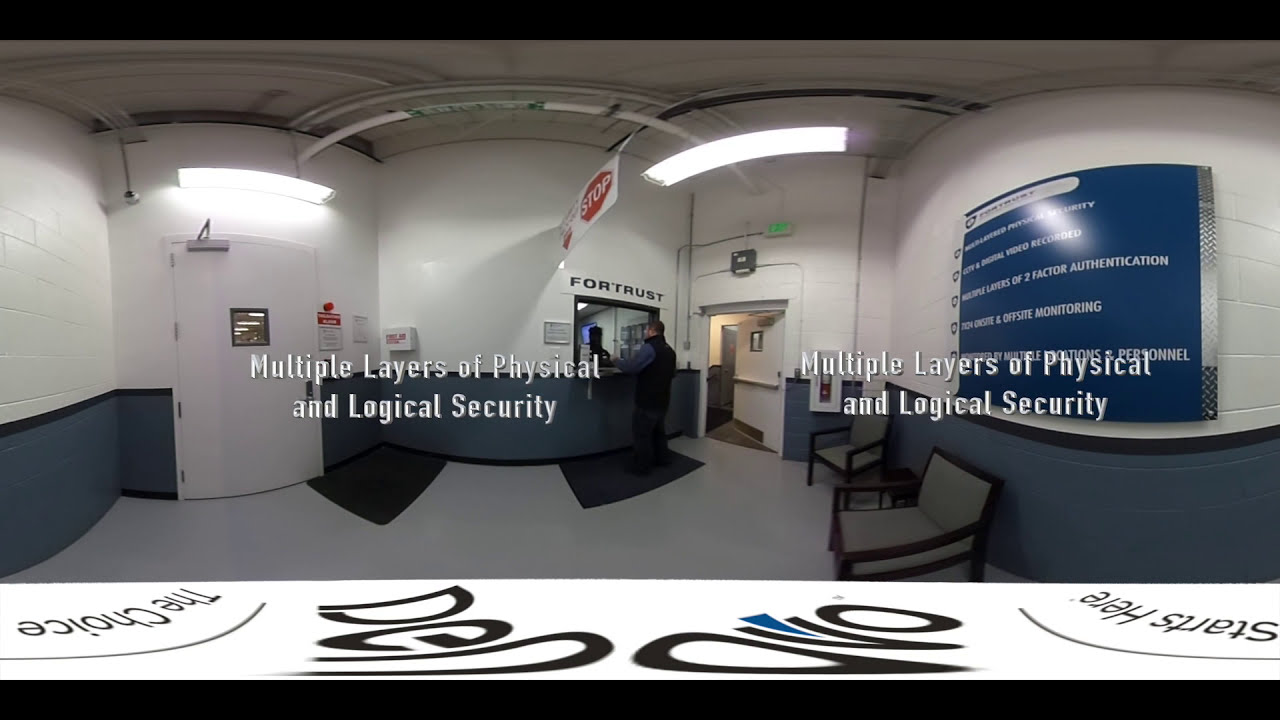The image depicts a panoramic view of an indoor security checkpoint or fortified area, possibly taken with a 360-degree camera, resulting in some warping of the proportions and curving of normally straight lines. The room has five walls, with the floor being plain gray. The walls are distinctly two-toned, painted dark navy blue on the bottom half and white concrete brick on the top half. Centered within the image is a small service window above which there is a sign with the word "FORTRESS" in black capital letters and another white sign with a red STOP symbol. A man dressed in black with a blue shirt stands facing this window. To the left, a white door with a square window in the middle is visible, while the right side features another white door, slightly ajar, and a long blue and white sign with partially readable text. Gray and brown chairs are positioned against the wall beneath this sign. The image is overlaid with white 3D text reading "multiple layers of physical and logical security" on both the left and right sides, indicating the secure nature of the environment. The image also includes a black rectangle at the top and bottom, with a distorted white bar containing black and blue lettering, noting upside-down phrases like "the choice" on the left and "starts here" on the right.